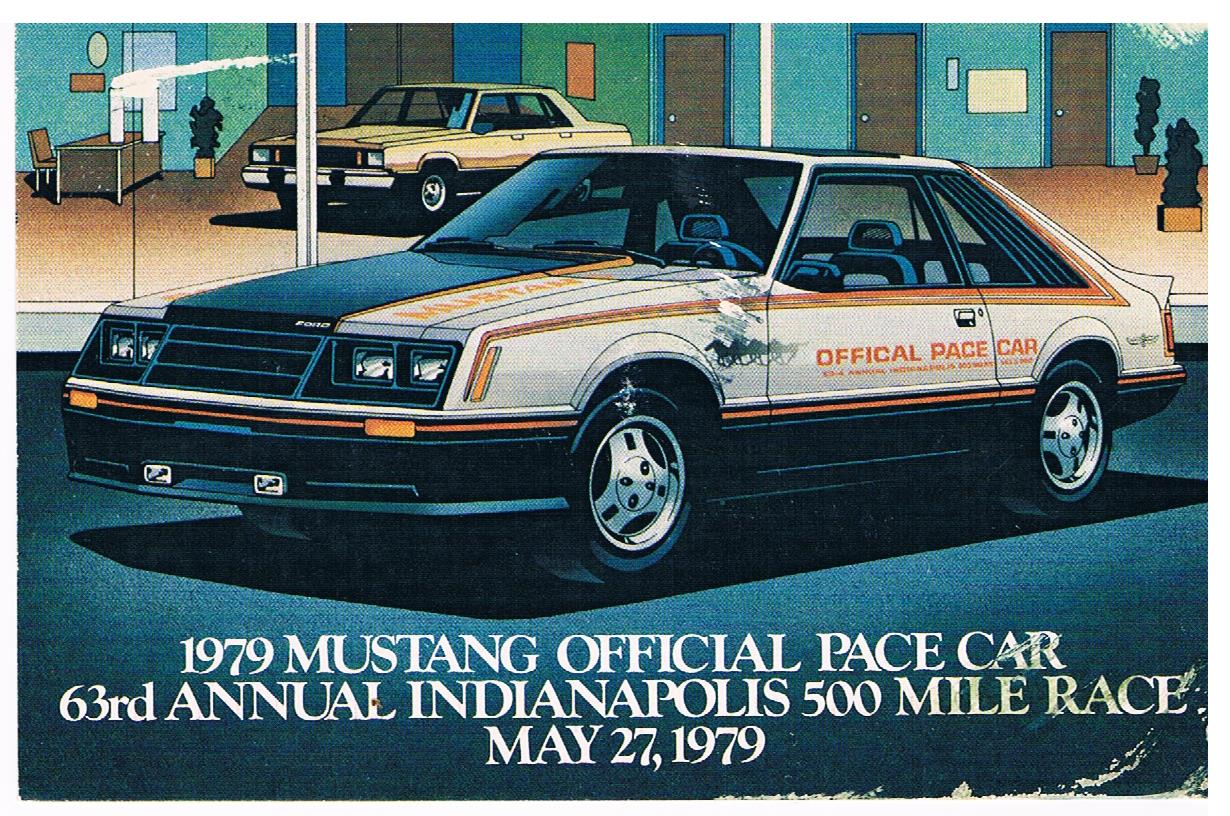The image depicts a hand-drawn advertisement showcasing the 1979 Mustang, the official pace car for the 63rd Annual Indianapolis 500 Mile Race, held on May 27th, 1979. The text, in bold white capital letters, stands out against a blue background towards the bottom of the illustration, providing event details. The car itself features a boxy, vintage design typical of the late 70s, with a black stripe down the center flanked by white sides adorned with orange stripes along the edges. The rims are detailed with a unique pattern of circular black dots and a triangular rim with double X rectangles at the center. The car, labeled "Official Pace Car", appears to be parked outside a showroom, visible through large glass doors behind it, adding a realistic touch to the cartoon-style drawing. The overall scene evokes the feel of a vintage magazine advertisement, complete with some scratches on the right side, indicative of its age and nostalgic value.